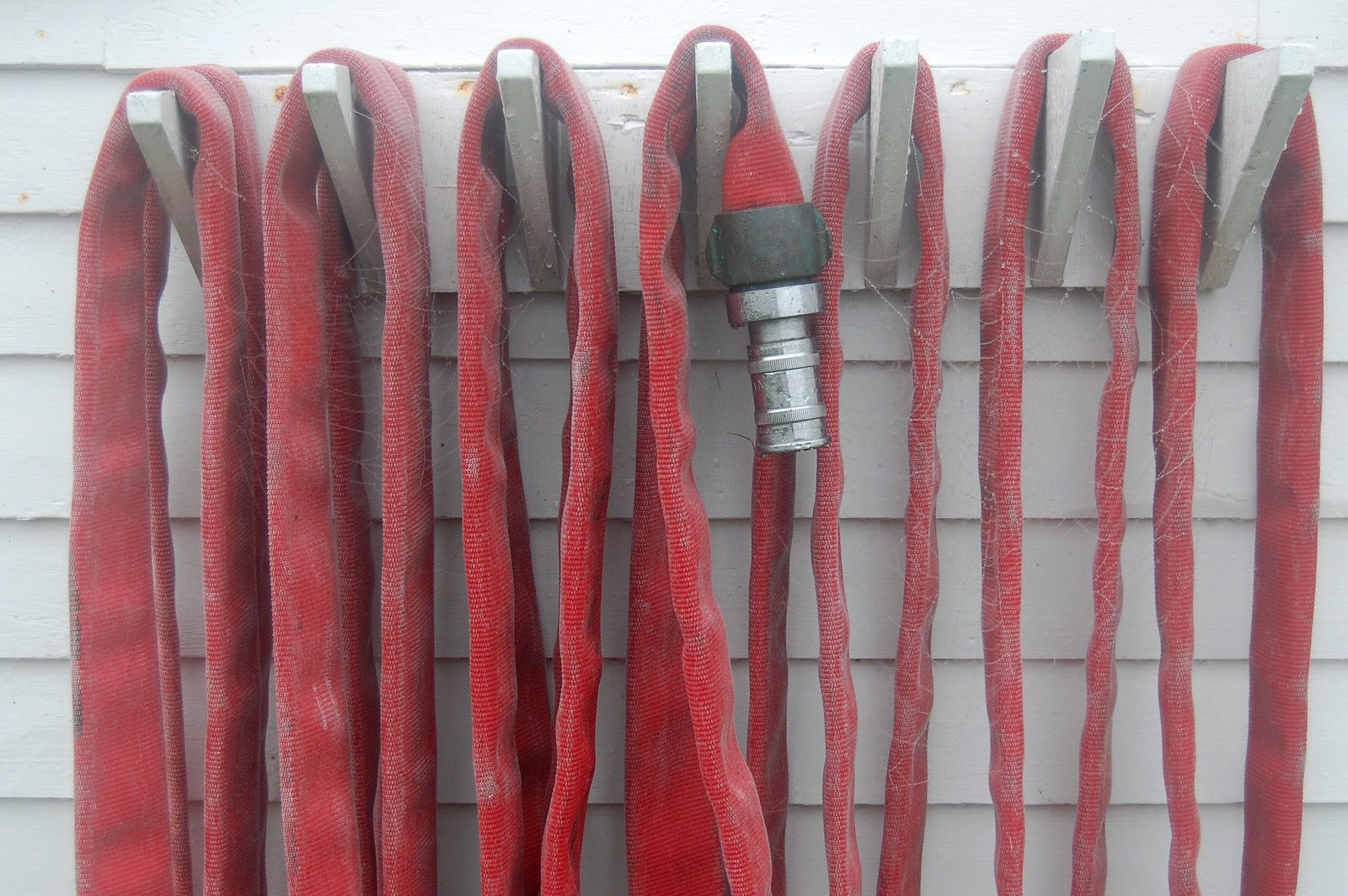The photograph is a detailed, color image taken indoors in landscape orientation, depicting a neatly organized display of seven red firefighter hoses. These hoses are mounted on a custom wooden rack against a white wall that seems to be tiled or use siding. The rack, which appears to be about three feet wide, has multiple triangular horizontal supports or slots designed to hold the hoses in place. While all the hoses are similarly arranged, the one in the center stands out with its prominent silver nozzle featuring a black rubber rim. The hoses vary in width, with some being noticeably thicker than others, and they are folded over to fit neatly on the supports. The background wall, composed of segmented, shingle-like white sections, has some visible dents, adding texture to the scene.